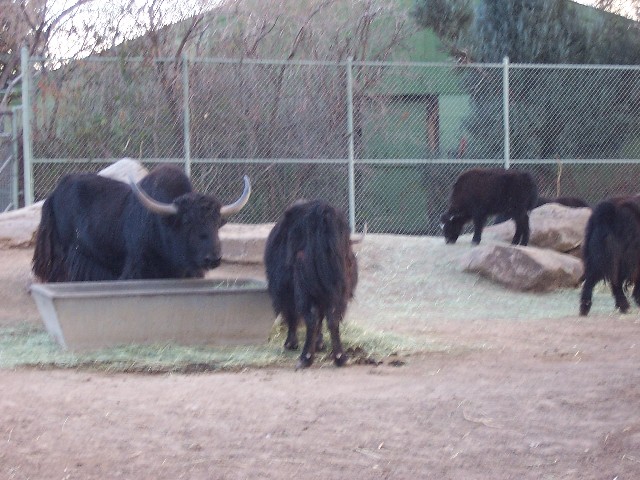The photograph captures a fenced-in farmstead featuring large, very hairy cattle akin to bulls or cows, predominantly black with shaggy coats and white or tan horns. In the center of the enclosure, a mix of grass and dirt surrounds a prominent feeding trough made of wood, stone, or similar material. To the left side, two of these cattle stand near the feeding trough, while to the right, additional cattle are positioned close to a cluster of brownish rocks. The backdrop includes a sparse arrangement of trees and a significant green metal building, indicating a rustic farm environment. The scene is mildly dreary, portraying both the practical elements of the animals' enclosure and hints of the larger farmstead beyond.